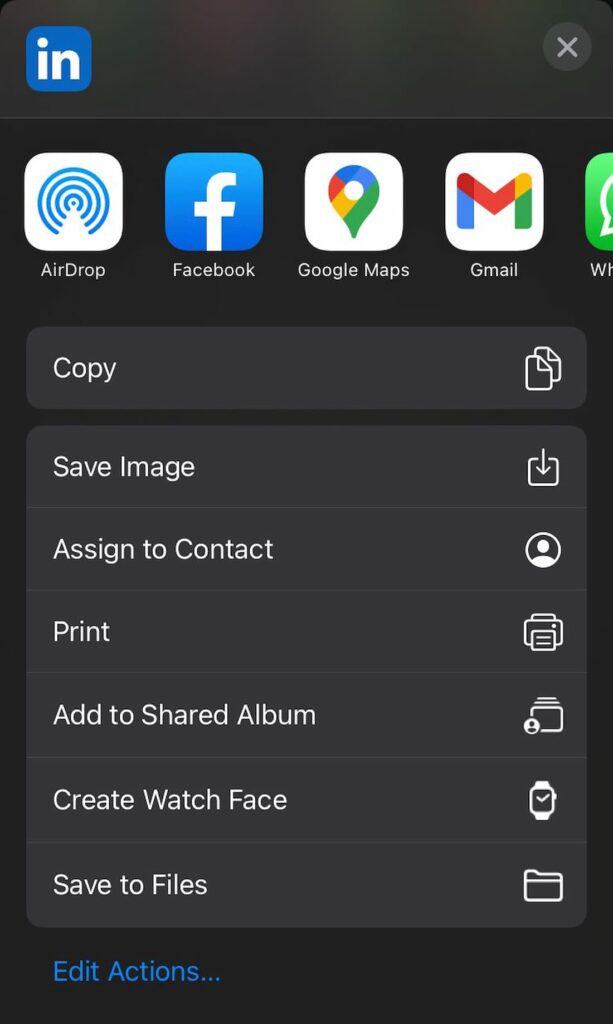This screenshot captures a share menu interface within the LinkedIn app, currently set to dark mode. At the top left corner, a blue square with the white letters "IN" signifies the LinkedIn logo. Below it, a grid of app icons is displayed, including AirDrop, Facebook, Google Maps, Gmail, and a partially visible WhatsApp icon. Directly below these icons, a series of actionable options are listed: "Copy," "Save Image," "Assign to Contact," "Print," "Add to Shared Album," "Create Watch Face," and "Save to Files," all in white font against the black background.

At the bottom left corner, a blue link labeled "Edit Actions" allows for customization of these options. On the top right corner, there is a light gray "X" icon to exit or close the menu. The device's dark mode setting is highlighted by the black background and white text, providing a clear and user-friendly interface for sharing content from the LinkedIn app.